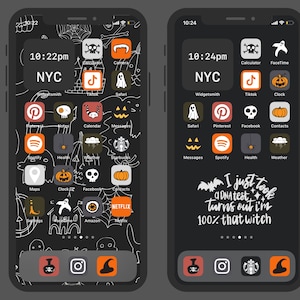The image displays two smartphones side by side, both featuring a Halloween-themed customization. The phones showcase a unique home screen setup where all the app icons are transformed into Halloween motifs, including pumpkins, skulls, a witch's hat, and a potion bottle. The icons are predominantly colored in shades of orange, white, and black, reflecting the spooky season. For instance, the Spotify app icon has turned orange, and the TikTok icon has also adopted the Halloween color theme. Some icons are entirely replaced with festive symbols – Starbucks, for example, is now depicted in black and white.

The background of the home screen is a deep black, adorned with intricate cobwebs and small spiders, enhancing the eerie atmosphere. A central widget displays the time as 10:22 PM and the location as NYC, indicating the current time and place.

On the phone to the right, there’s a cursively written phrase partially visible, which reads, "This is 100% that witch." This reinforces the Halloween theme with a playful twist. The overall setting of the image appears against a simple gray background, which contrasts with the vibrant, spooky customization of the phone screens.